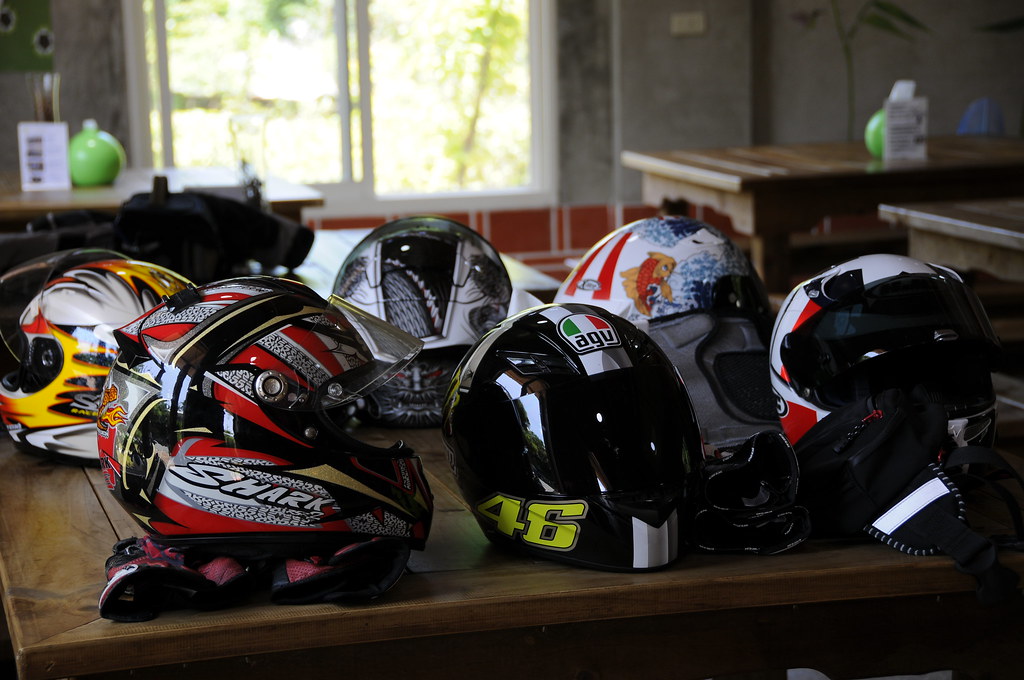The photo captures the interior of a room, potentially a garage, featuring several tables and a concrete wall with a window. Central to the image is a brown wooden table displaying six distinct motorcycle helmets, each adorned with various colors, designs, and logos. The forefront of the table presents three helmets: a red and white one branded 'Shark,' a black helmet with a white stripe and a yellow number '46,' and a third in red and white. Behind these sit three more: a mix of yellow, red, and white helmets, each with unique details, including cartoon figures and intricate patterns. All helmets have visors, suggesting they are geared for motorcycle or race car use. In the background, other empty tables and a glimpse of trees outside the window complete the scene.